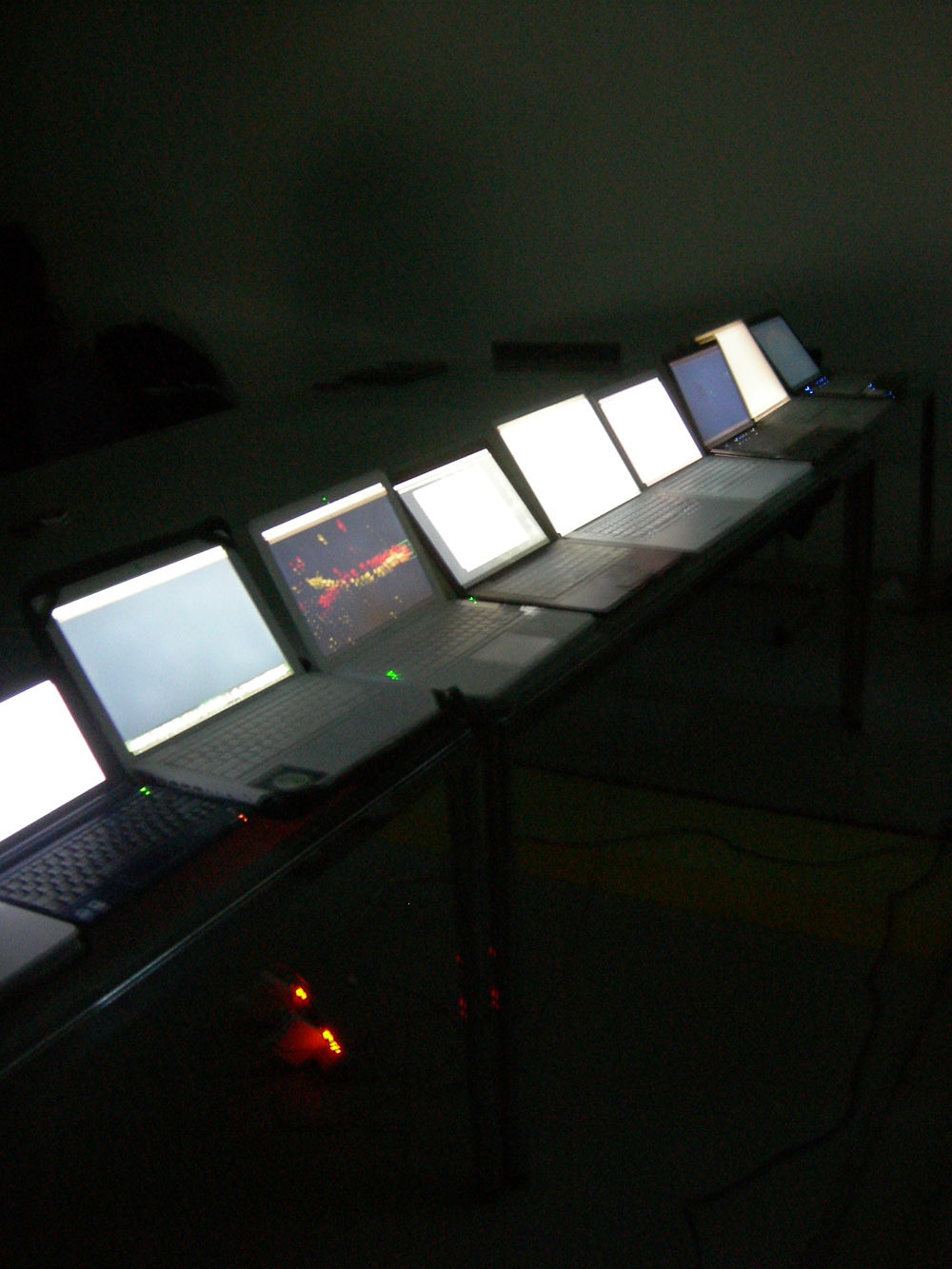In a dimly lit room, two expansive gray-brown tables with black legs stretch across the space. On these tables is a diagonal row of nine open laptops, their screens illuminating the dark setting. The laptops vary in size and color—silver, black, and gray—and are secured with a cord running beneath the tables. A large power strip with glowing orange lights lies under the table. Most screens appear blank, but the third laptop's display stands out with a vivid red and yellow twisty line against a dark background, hinting at a space-themed image. Three unoccupied chairs line the far side of the setup, adding to the stillness of the room. The barely visible furniture and cords set a quiet, almost eerie scene under the subtle glow of the laptop screens.